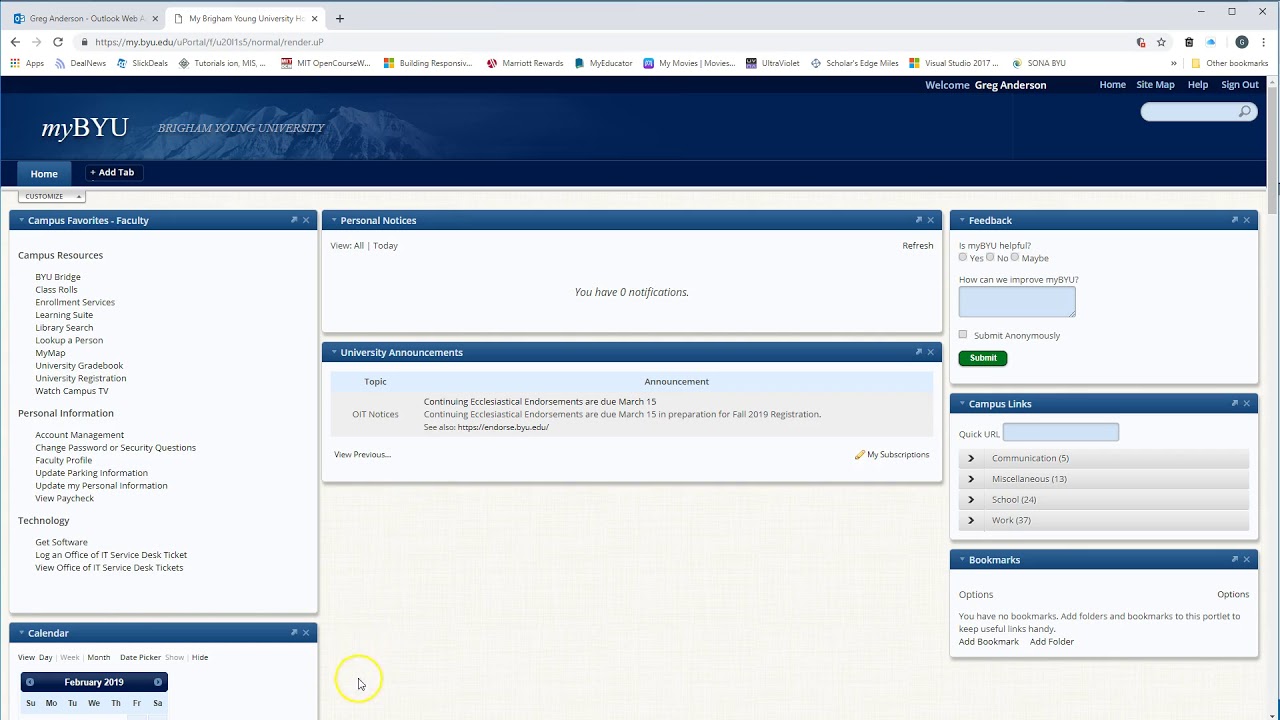**Detailed Caption:**

The image depicts the personal dashboard of Greg Anderson on the Brigham Young University (BYU) Outlook Web platform. His screen showcases various navigational options and tabs, reflecting a fully customized and resource-rich interface for students and faculty.

The diverse array of sections and tools available on Greg's dashboard includes links to campus resources, faculty services, and personal account management. Specifically, there are tabs for 'Campus Favorites', 'Faculty Profiles', 'Learning Suite', and 'Library Search'. There are also sections for 'Enrollment Services', 'Classrooms', 'BYU Bridge', and 'University Gradebook'. A 'Calendar' widget is visible, showing the dates for February 2019, enabling users to view days, weeks, and month details, with a visible cursor hovering over a yellow circle.

Additional references on the page include curated lists of resources like 'MIT OpenCourseWare', 'Building Responsive Web Design', 'Visual Studio 2017', 'My Movies', 'Slick Deals', and 'Merit Rewards'. The presence of technical support options is evident with links to the 'Office of IT Services', 'Software Login', 'Test Ticket View', and 'Technology Services'.

Greg's dashboard also appears to offer personal management features like 'Account Management', 'Change Passwords', 'Security Questions', and 'Park Information'. The welcome segment confirms the user as Greg Anderson, with options to navigate home, add tabs, or sign out. A magnifying glass icon signifies a search function, complementing the comprehensive design of the BYU portal to enhance the user experience for their academic and personal needs. 

Overall, the image captures a highly functional and detailed overview of the BYU portal, tailored for effectively navigating the university's digital offerings.